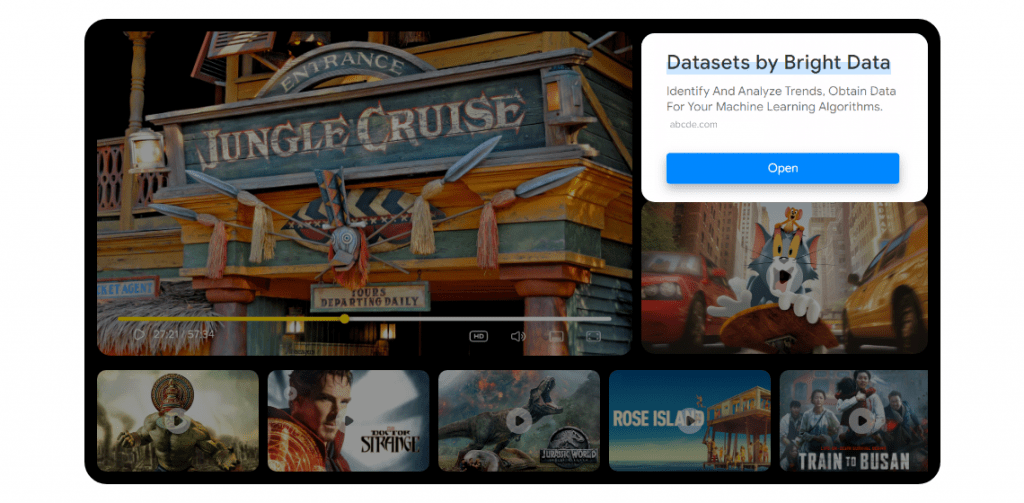This image captures the interface of a streaming website displaying an array of movies, prominently showcasing data sets supplied by "Bright Data." Below this, there is a tagline reading, "Identify and analyze trends, obtain data for your machine learning algorithms," along with a button labeled "Open." 

The visible movie thumbnails include the following:

1. **"Jungle Cruise"** – A screenshot depicting the adventurous scenes typical of the movie.
2. **"Lewis Tompkins Sherry"** – Featuring a still presumably from this dramatic film.
3. **"Doctor Strange"** – Showcased with a notable image from the Marvel superhero movie.
4. **"Jurassic World"** – Highlighting a thrilling moment from the dinosaur-centric film.
5. **"Rose Island"** – An image capturing the essence of this unique narrative.
6. **"Train to Busan"** – Displaying a tense scene from the popular zombie apocalypse thriller.

All text elements, including movie titles and descriptions, are displayed in a slightly dark gray hue, providing contrast against a bright white background, which enhances readability and visual clarity.